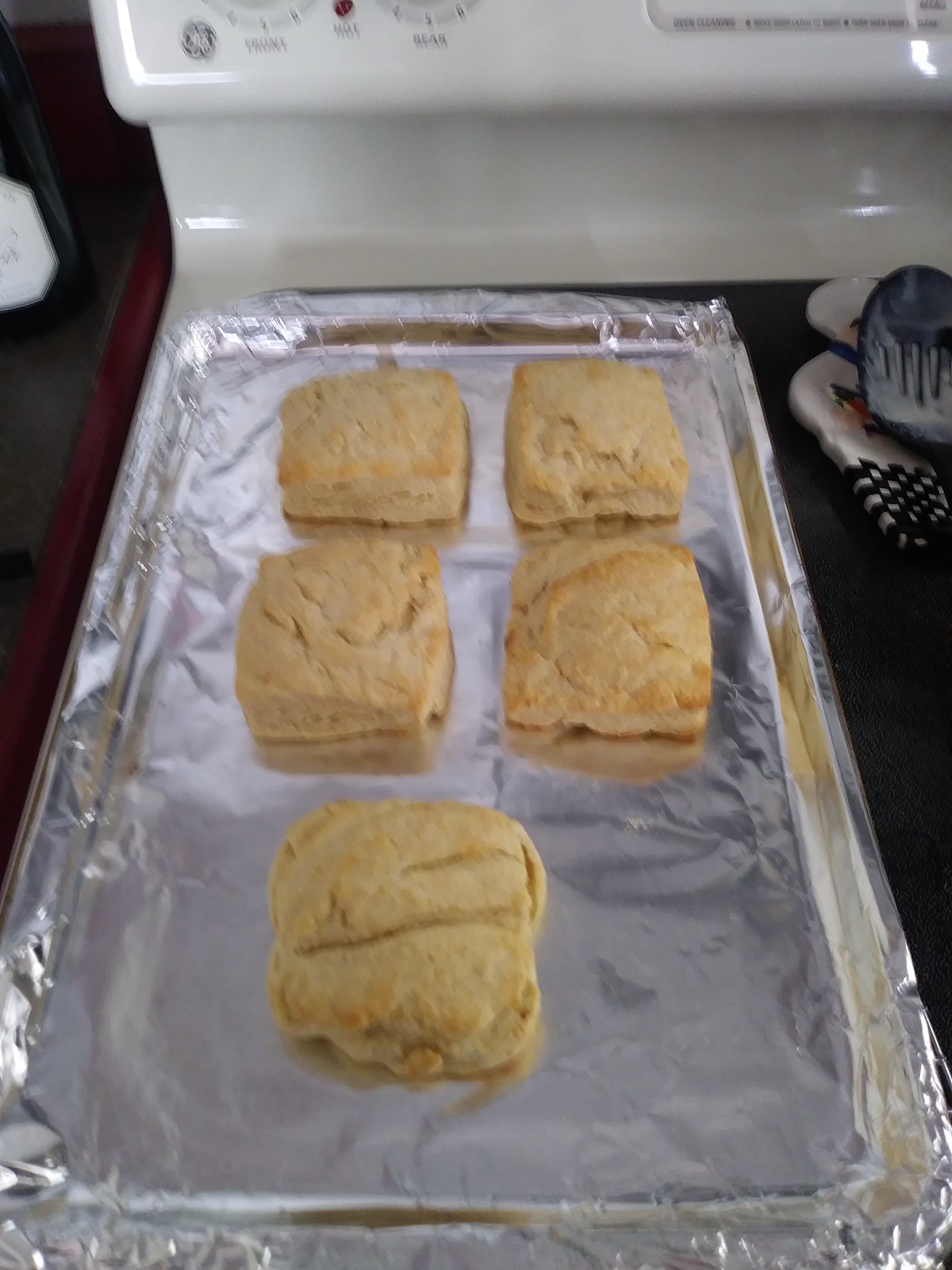In the image, you can see a white General Electric stove positioned on the right, partially visible with a red indicator light and two control knobs on the left. A black countertop with a red border lies to the left of the stove. On the stove's surface, there is a baking sheet wrapped in aluminum foil. This sheet holds five square, light golden brown biscuits arranged thoughtfully in two rows of two and one at the bottom. These homemade, crumbly biscuits appear thick and substantial. Additionally, a slotted spoon can be seen on the stove’s surface and, on the far left side, a glimpse of a white and black checkered wrist oven mitt is visible along with some faint writing in the image’s upper right corner.